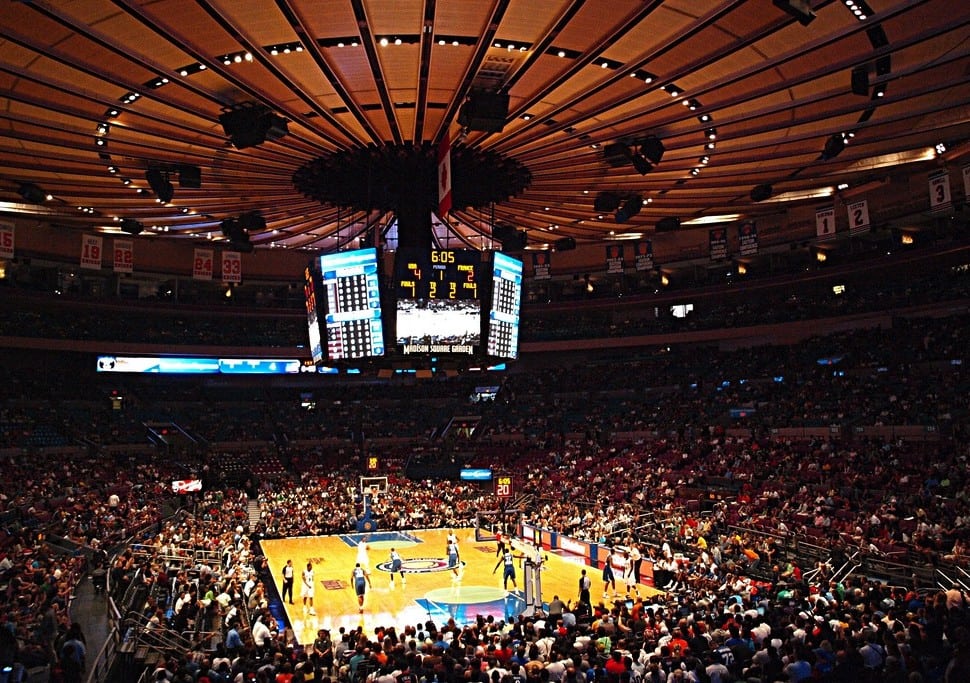The image presents a detailed aerial view inside a bustling basketball arena, likely Madison Square Garden, given the distinctive brownish-wooden patterned roof resembling a fan and housing thousands of spectators. The court beneath is bathed in bright white lighting and features a yellowish-brown surface complemented by blue accents. The scene captures a professional basketball game, with one team likely the New York Knicks in white uniforms and their opponents in blue. The focal point over the court is a massive scoreboard surrounded by six giant monitors, displaying a score of 4-2 with 6:05 left on the clock, along with stats that are too small to discern. Adding to the international ambiance, a Canadian flag hangs prominently from the ceiling. The crowd, nearly filling every seat, contributes to an electric atmosphere, colored in an array of black, white, brown, gray, blue, yellow, red, orange, and pink. From this vertical perspective, you can clearly see one goal at the front and another in the back, capturing the intensity and scale of the event.